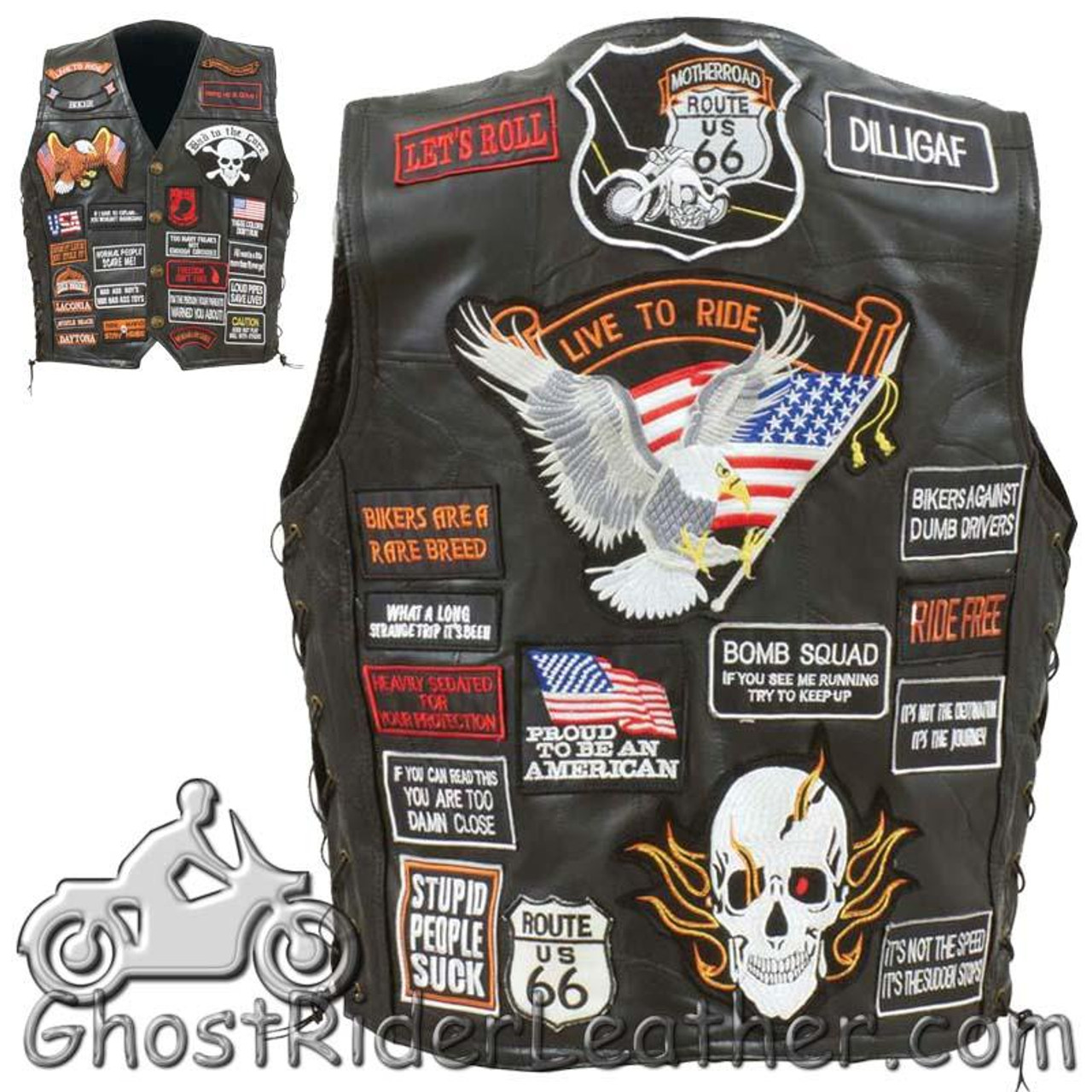The image showcases a black, sleeveless motorcycle leather vest, prominently displayed from the back with a smaller inset of the front in the top left. The vest is adorned with an eclectic array of approximately 16 to 17 patches, depicting various generic biker phrases and symbols that seem more commercially driven than authentic to any specific biker group. 

Dominating the center back of the vest is a large patch of an eagle clutching an American flag, with the words "Live to Ride" emblazoned above. Surrounding this centerpiece are numerous smaller patches, such as "DILLIGAF" in white on the top right, "Let's Roll" in red on the top left, "Stupid People Suck" in white on the bottom left, and "It's Not the Speed, It's the Sudden Stops" in white on the bottom right. Additional patches include sayings like "Ride Free," "Bikers Against Dumb Drivers," "Bomb Squad - If You See Me Running, Try to Keep Up," and "Mother Road Route U.S. 66" with an image of a white motorcycle.

At the bottom of the image, a logo for ghostriderleather.com features a metallic stencil of a person on a motorcycle, indicating that this vest is likely a commercial product rather than an authentic piece of biker gear. The overall impression is of a costume piece, made for those looking to mimic biker culture without truly belonging to it.